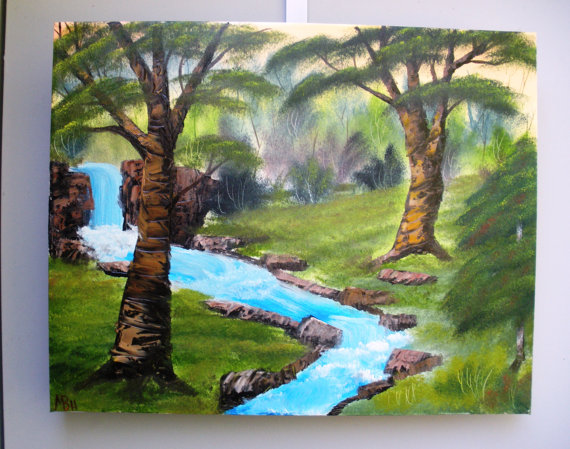This image is of a detailed, playful drawing that captures a serene, tropical scene. Dominated centrally by a vivid blue river, the water starts as a small waterfall nestled between cliffs on both the right and left. The river cascades down from the middle-left edge and then gracefully curves to the right before angling back left to the middle bottom of the drawing. On the left bank of this meandering river stands a prominent tall tree amidst lush grass, while the right bank mirrors this with additional grassy terrain, another tall tree, and a scattering of bushes. The background includes more trees, some of which resemble tropical varieties, adding to the rainforest vibe. Surrounding the water are various boulders and cliffs, creating a rich and naturalistic landscape. The picture itself, likely a watercolour or an intricately done crayon piece, is set on a white wall, giving the entire scene a neat, framed appearance.